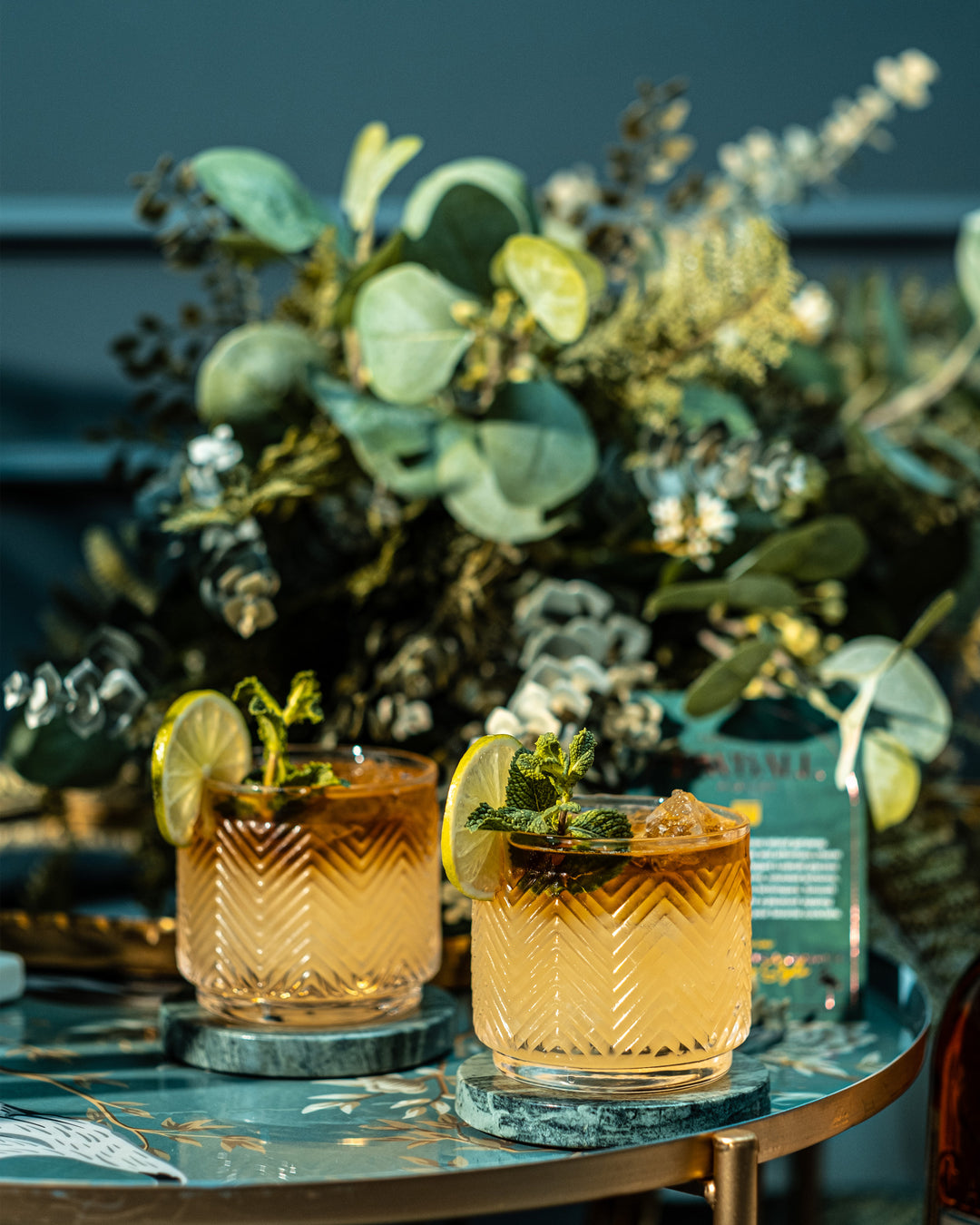This vertical rectangular image depicts a meticulously arranged scene focused on two vintage cocktail glasses situated in the foreground. Each glass is a few inches tall, clear, and adorned with a distinctive raised wavy pattern, suggesting a design reminiscent of the mid-20th century. They sit on round, teal coasters that blend harmoniously with the table surface beneath them—a light teal tabletop embellished with delicate white floral patterns and bordered with a dark gold trim. 

The cocktails within these glasses display a gradient of color, from light yellow at the base to a darker brown at the top, possibly hinting at a splash of cola—a characteristic element of a Long Island Iced Tea. Each glass contains an ice cube, a piece of lemon, and a surprising garnishment of broccoli, adding a unique splash of color along with a slice of lime gracing each rim. The backdrop of the photo shows a slightly blurred teal wall adorned with vibrant green plants that include hints of white and blue, contributing to the image's verdant theme. The scene is completed by the hints of dark gold from the table's legs and trim, creating a complementary and well-balanced color palette.